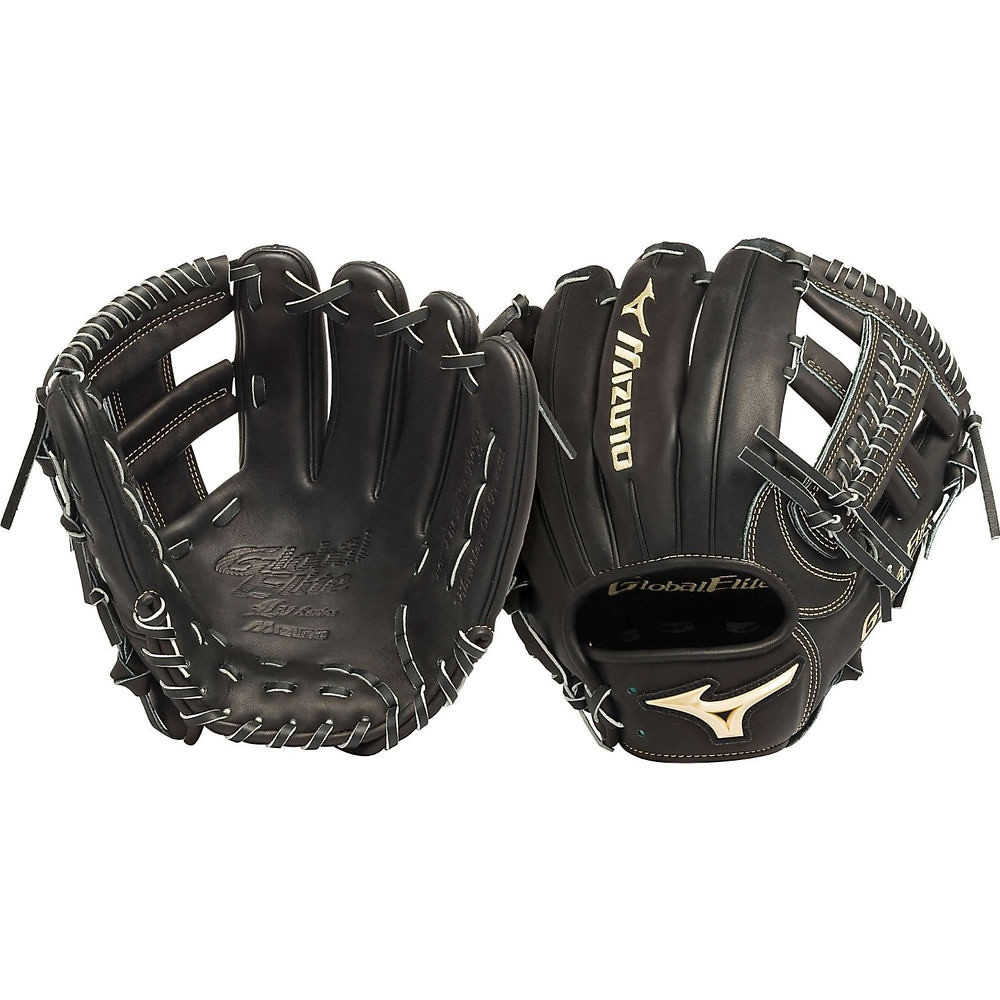This close-up photograph showcases a pair of Mizuno baseball gloves against a clean, white background, resembling an image from a retailer's website. The gloves, predominantly black with striking white stitching, are positioned with one glove displaying its palm and the other showing its back. The left glove's palm, oriented outward, features an embossed "Global Elite" logo. The right glove presents the back, with "Mizuno" prominently printed on the middle finger in bold white letters, accompanied by a distinctive sideway "Y" or swish-like logo. The wrist strap of the glove also bears another symbol, maintaining brand consistency across both gloves. This meticulously detailed image highlights the craftsmanship and branding of the Mizuno baseball gloves, emphasizing their premium quality and design.